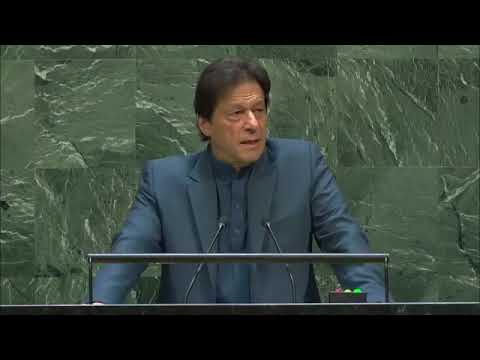The image depicts an older, light-skinned man standing at a podium, delivering a speech or being interviewed, with two slender, bent microphones positioned in front of him. He is dressed in a dark green suit with a hint of blue, complemented by a matching blue button-up dress shirt. The background consists of large square tiles in various shades of green, including sage and darker greens with white lines, giving the impression of a marble wall. The overall setting appears to be indoors, possibly a formal or government environment. The image is framed by black borders at the top and bottom. The man, positioned directly at the center, looks slightly to his right, possibly addressing an audience or group of people. There is no visible text in the image, but the backdrop features a mosaic of colors including shades of green, blue, yellow, red, and brown, adding depth to the scene.